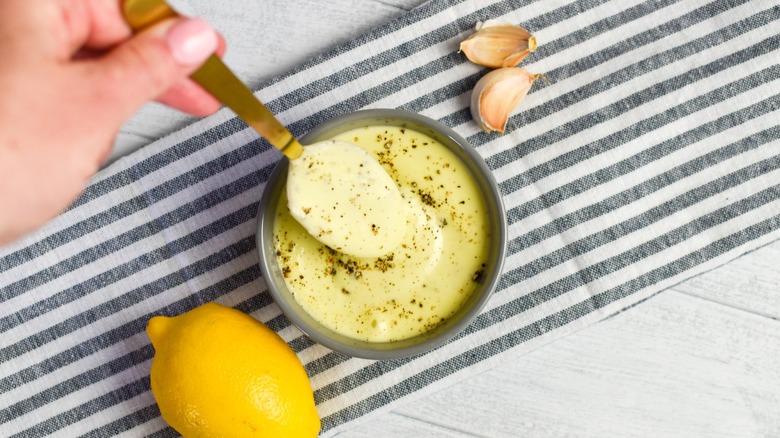This overhead landscape photograph captures a culinary moment with precise detail. Central to the image is a small, circular, grey stoneware bowl holding a creamy white sauce speckled with green flakes, possibly herbs or spices. A left hand, with pink-painted fingernails suggesting a woman's hand, holds a brass spoon poised just above the sauce, either dipping in or lifting out. This scene unfolds on a grey and white striped kitchen towel, resembling a seersucker suit pattern. To the left of the bowl sits a whole lemon, while to the right are two cloves of garlic. The setup rests on a white tiled or wooden surface, adding a clean backdrop to the focused preparation.